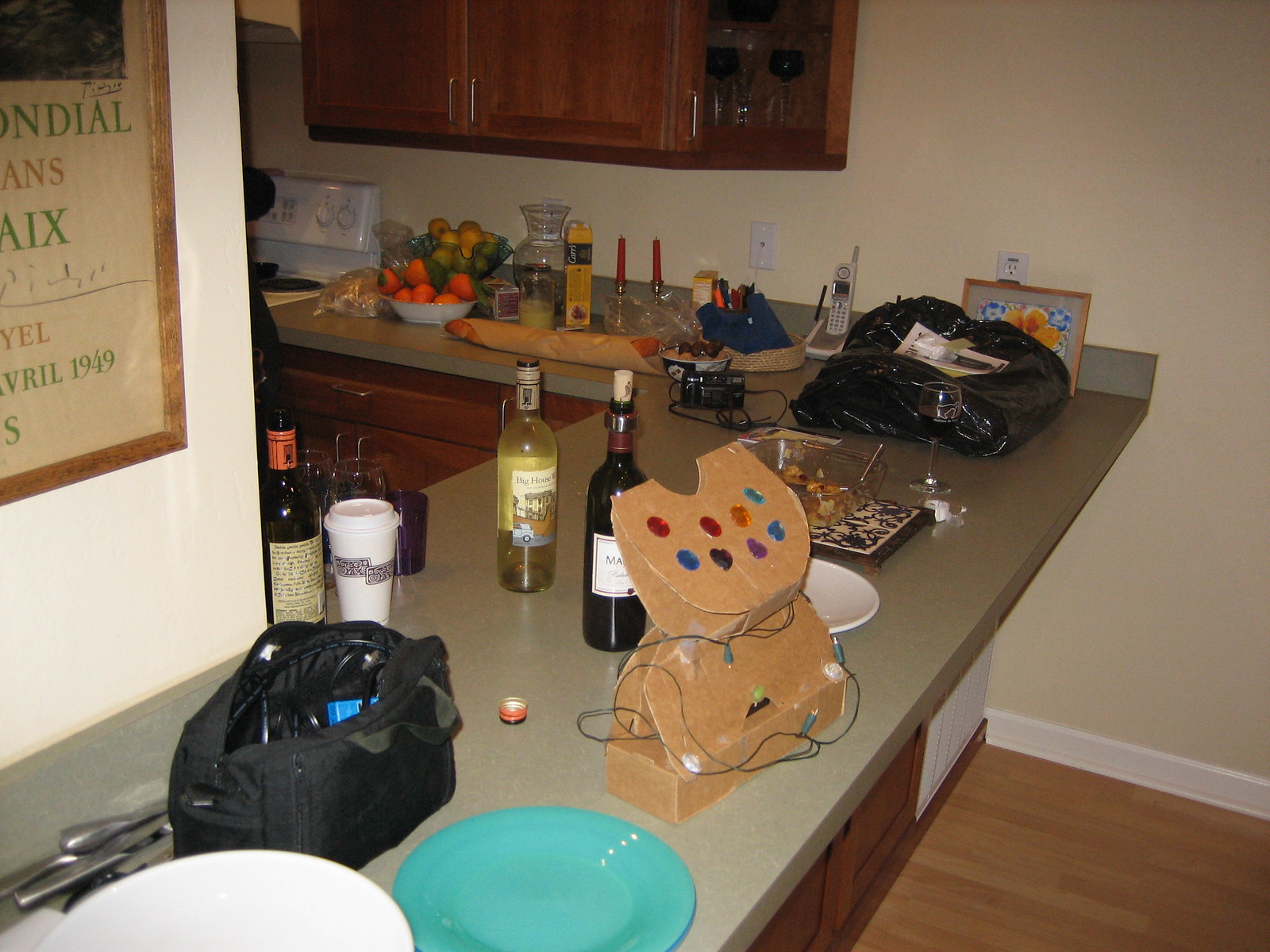This image captures a cozy, multifaceted room that seamlessly blends the kitchen and living room areas. A prominent feature is a multifunctional table that acts as a divider between the two spaces. The table, which has a brownish top and wooden bottom, extends to the wall where it makes a right turn, continuing further into the kitchen area.

On the table, a variety of items are scattered, including plates, a fabric bag filled with miscellaneous items, a cardboard item secured with tape, and strings of Christmas lights. There are also several bottles of alcohol adding to the eclectic array.

Closer to the kitchen section of the table, there's a loaf of bread and a couple of bowls filled with fruit. Above this setup, within the kitchen, is a set of wooden cabinets. One of the cabinet doors is open, revealing an assortment of drink glasses.

The flooring in the kitchen area is a warm, wooden surface, while the walls boast a soothing beige color. On the right side of the room, a white wall serves as a backdrop for a decorative poster, adding a touch of personality to the space.